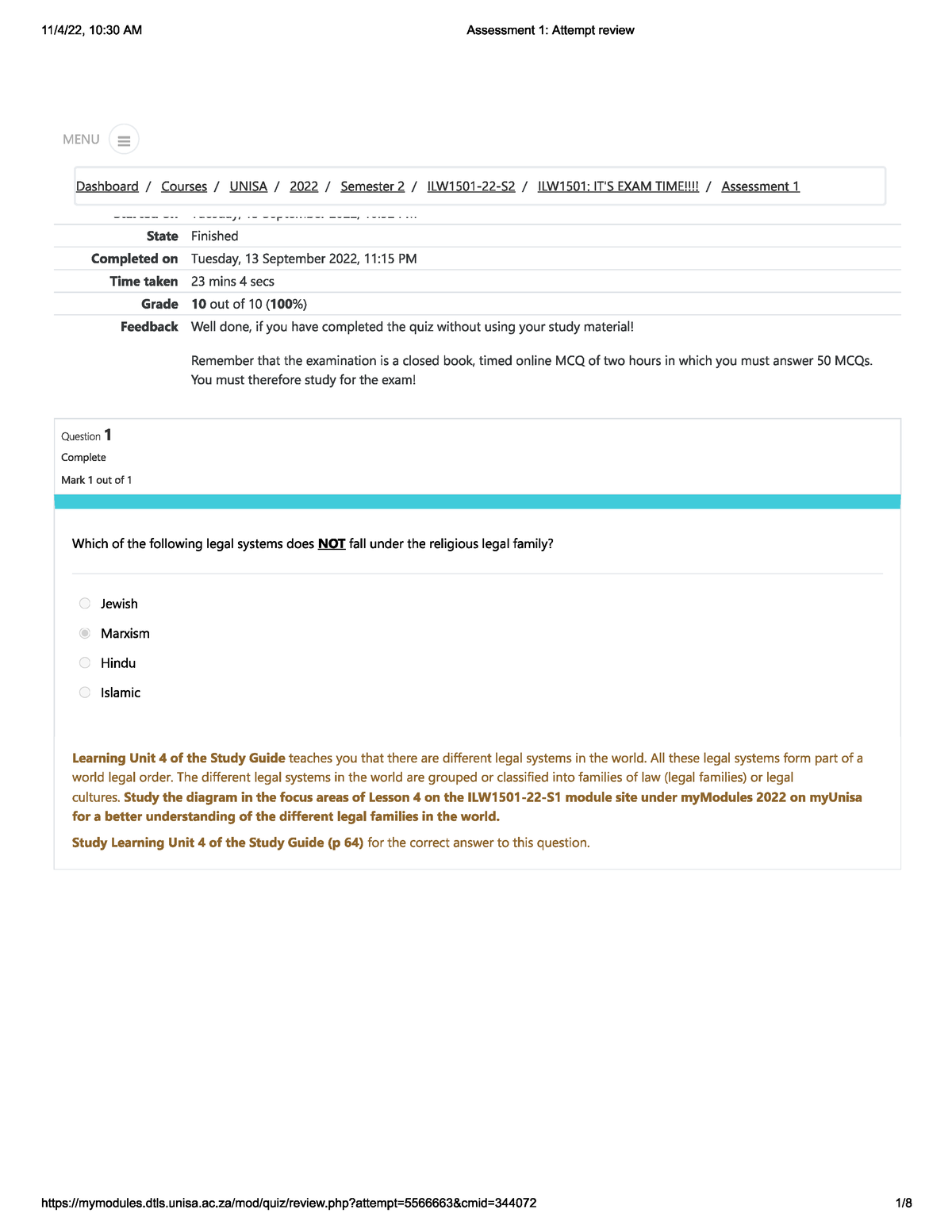Here's a detailed and cleaned-up caption for the described image:

---

The image displays a webpage with various sections of text and navigation elements. The content is framed in a square format, and it is impossible to discern the device being used to view the page. 

In the top left corner, the date "11/4/22" and the time "10:30 AM" are clearly displayed. To the right, the title "Assessment 1: Attempt Review" is prominently positioned. Near the top right, there is a lighter gray menu icon featuring three horizontal lines.

Immediately below, a navigation breadcrumb trail appears, reading: "Dashboard / Courses / UNISA / 2022 / Semester Two / ILW1501-22-52 / ILW1501: IT'S EXAM TIME!!!! / Assessment 1," with each element underlined.

The next section, labeled "State," indicates the following completion details: "Finished, Completed on," "Time Taken," "Grade: 10 out of 10." A feedback note is provided: "Well done if you've completed the quiz without using your study material." Additional instructions are given, emphasizing that the examination is a closed book, timed online multiple-choice quiz (MCQ) to be completed in two hours, consisting of 50 MCQs. Students are reminded to study for the exam appropriately.

Question 1 shows a complete status with a score of "1 out of 1." The question is, "Which of the following legal systems does not fall under the religious legal family?" with the correct answer being "Marxism." 

Additional learning resources are referenced in brown text, guiding students to Learning Unit 4 of the study guide. It explains that various legal systems in the world are classified into families of law, and advises looking at the diagram in the "Focus Area of Lesson 4" on the ILW1501 module site under "myModules 2022" on "myUNISA." The students are also encouraged to study page 64 of Learning Unit 4 in the study guide for the correct answer to the question.

---

This provides a detailed and structured view of the webpage content, emphasizing important elements and instructions for the student audience.